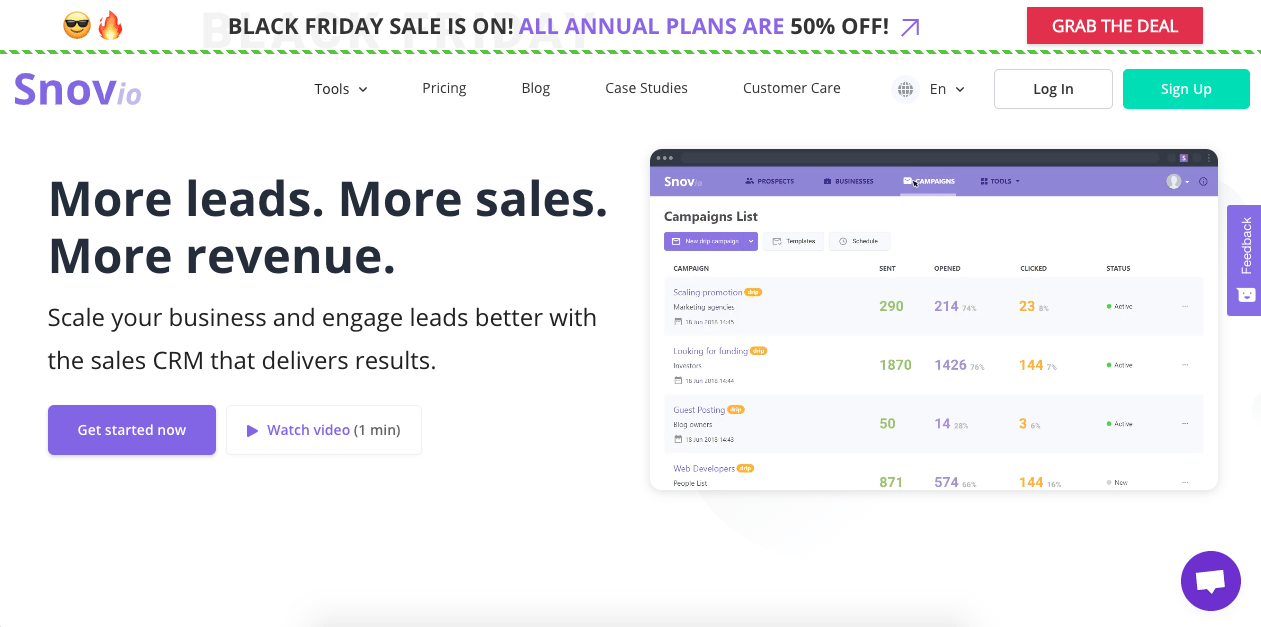This image is a screenshot from the website SNOVIO, as indicated by the name "SNOVIO" prominently displayed in the upper left-hand corner. Above the SNOVIO logo, there is a highlighted announcement separated from the rest of the site by a thin green line that stretches horizontally across the top. This section announces a Black Friday sale, stating: "Black Friday sale is on. All annual plans are 50% off." Additionally, there is a call-to-action button labeled "Grab the deal."

Below this announcement, the website features a main menu with the following options: Tools, Pricing, Blog, Case Studies, Customer Care, and a language selection currently set to English. To the far right of this menu, there are two buttons for user actions: "Login" and "Sign Up."

Dominating the main section of the page, bold text reads: "More leads, more sales, and more revenue," followed by a subheading: "Scale your business to gauge leads better with the sales CRM that delivers results."